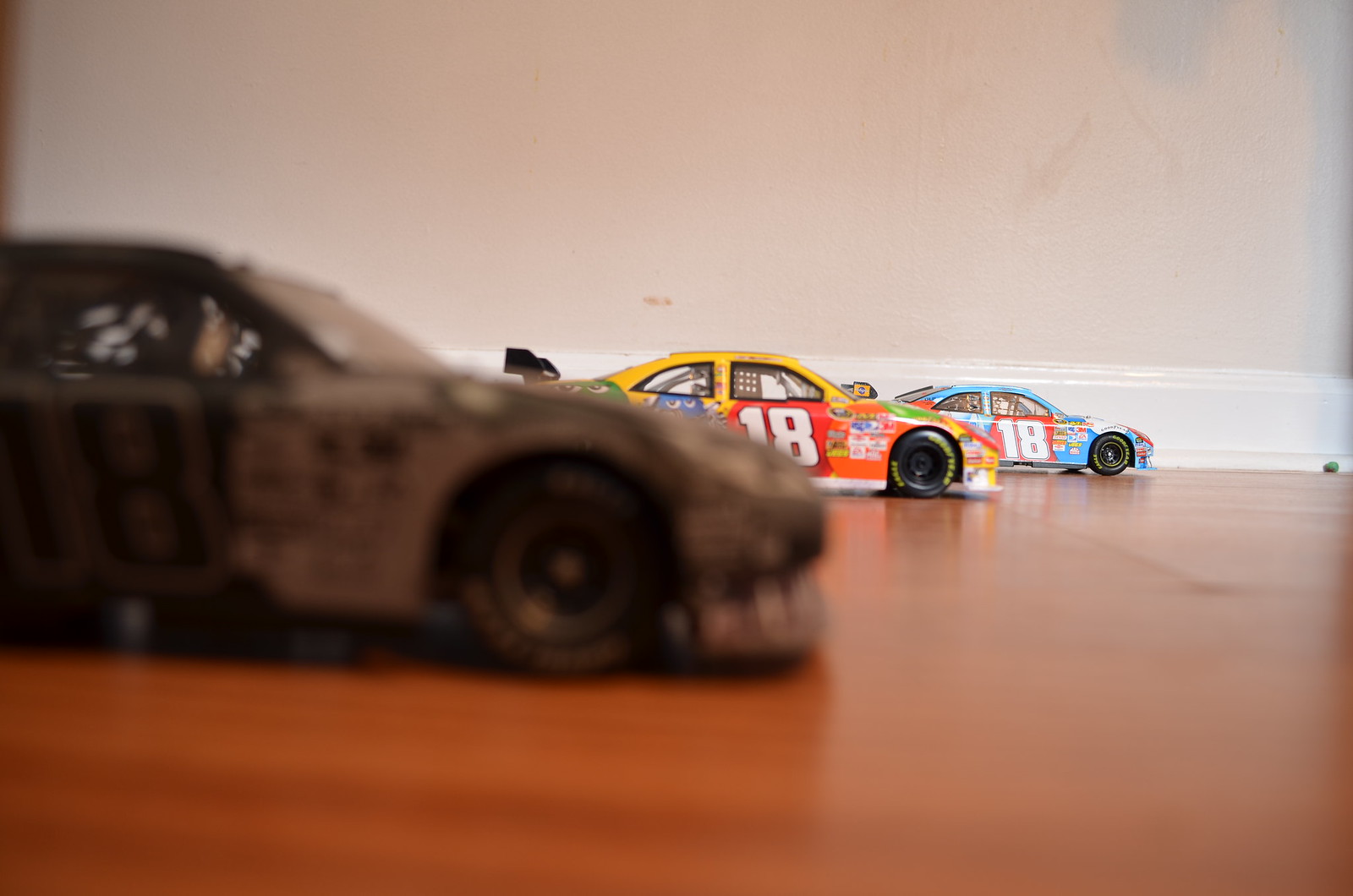This detailed indoor scene captures a close-up of three toy NASCAR race cars arranged on a wooden floor. The camera is positioned at a low angle, giving the impression that the matchbox-sized cars are full-sized vehicles on a racetrack. The backdrop includes white baseboards, accentuating the miniature scale of the cars.

The cars sport detailed designs with bold numbers and logos, typical of stock cars. The nearest toy car—a gray and black model—is out of focus due to the camera's perspective. The middle car, brightly colored in yellow with various designs and logos, stands out. The farthest car is predominantly light blue with red accents. All cars bear the number 18 and feature netting and roll cage bars, emphasizing their authentic NASCAR appearance. They are staggered along the floor, adding a dynamic sense of movement to the scene.